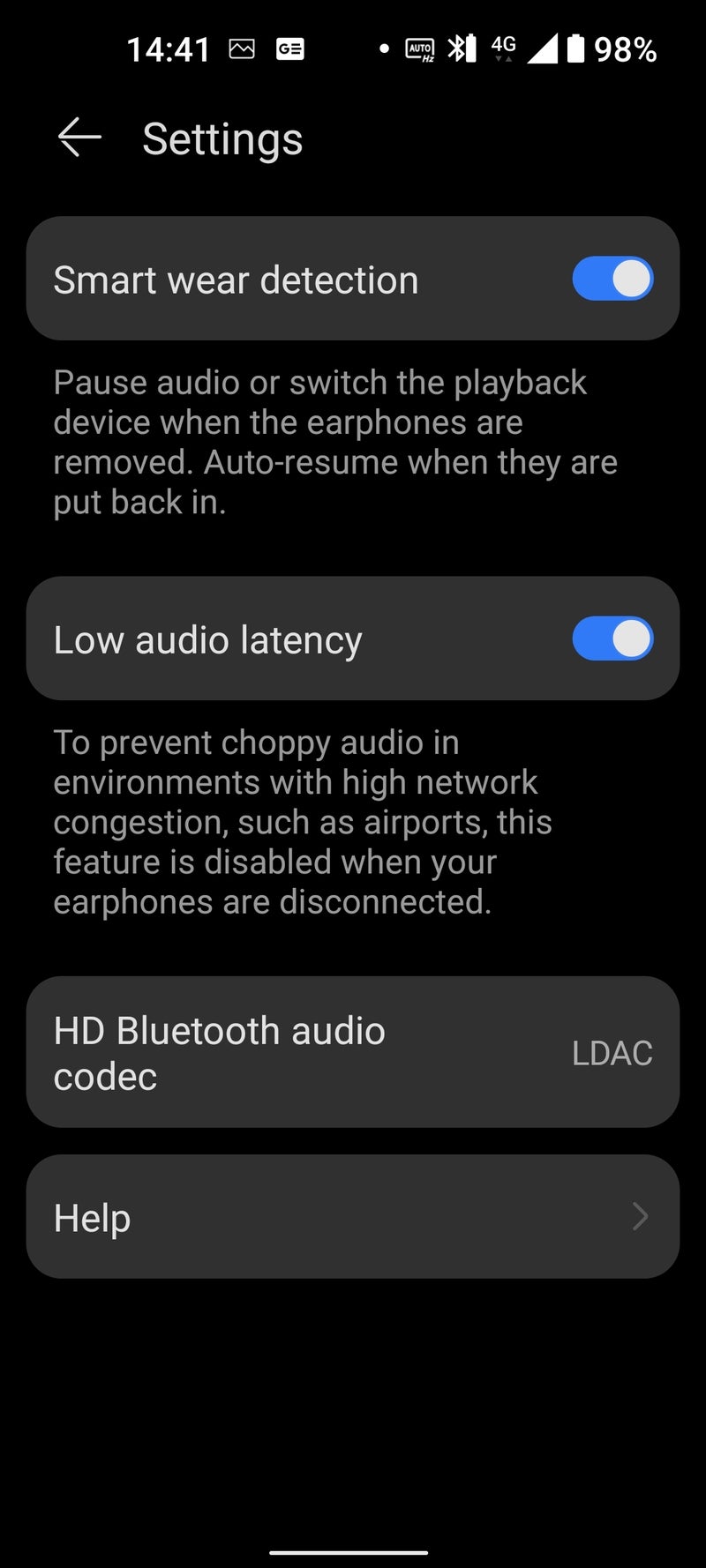This is a detailed screenshot from a smartphone, taken in portrait orientation. 

- At the very top of the screen, the status bar displays the time in military format as 14:41. 
- Next to the time is an unnamed box icon, accompanied by another indistinct icon that can't be clearly identified. 
- This is followed by a small white dot, another unidentified icon, the Bluetooth icon, the 4G icon, and the signal bar, which is fully filled. 
- The battery percentage next to the battery icon reads 98%.

Beneath the status bar:

- On the left is a back arrow pointing to the left, labeled "Settings." 
- Below this header is a rectangular box labeled "Smart Wear Detection," which is toggled on. 

Underneath "Smart Wear Detection":

- There is a description: "Assist pulse audio or switch to playback device when the earphones are removed. All resume when they are put back in."

Following this description:

- Another rectangular box is labeled "Low Audio Latency," and it is also toggled on. 
- Next to this label, there's a note: "To prevent choppy audio in environments with high network ingestions such as airports, this feature is disabled when your earphones are disconnected."

Further down:

- There is another rectangular box labeled "HD Bluetooth Audio Codec," with "LDAC" indicated on the right side of this box.
- Lastly, another rectangle contains the label "Help," with an arrow pointing to the right on its right-hand side. 

This screenshot appears to be from a smartphone's settings menu, specifically related to audio and Bluetooth configurations.